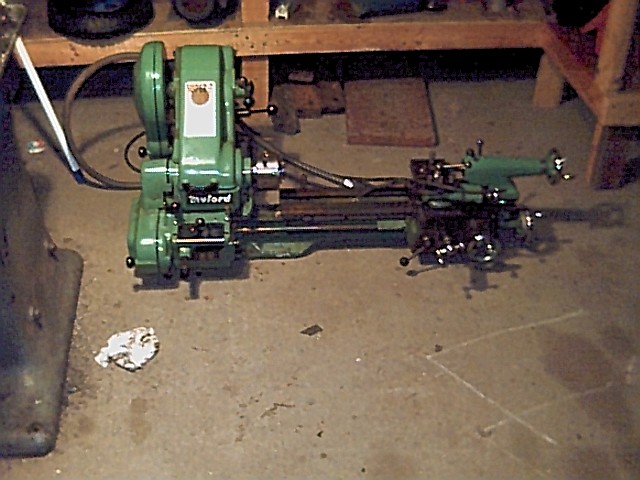The image captures a cluttered garage or workshop with a prominently featured piece of green machinery positioned on a dirty, debris-covered concrete floor. The floor is marked by scratches, dirt, and what appears to be a crumpled piece of paper. To the left of the machinery, there is another piece of equipment with a silver metallic frame, including protruding bolt ends and a supporting leg with a black foot. There is a prominent large green apparatus on the left side of the machinery, extending into a brown section, and then a smaller green part on the right side. The apparatus includes multiple levers, knobs, and cables, some of which are black and possibly a plug-in cord. Highlights include a white label and a gold circular emblem on the upright green segment. Surrounding the machinery are shelves and a wooden table, laden with indeterminate items and darker materials, possibly bricks tucked under the table. These shelves appear rusty and support scattered unidentified objects. The scene hints at a busy, possibly neglected workspace, reflecting an environment where detailed work with machinery frequently occurs.